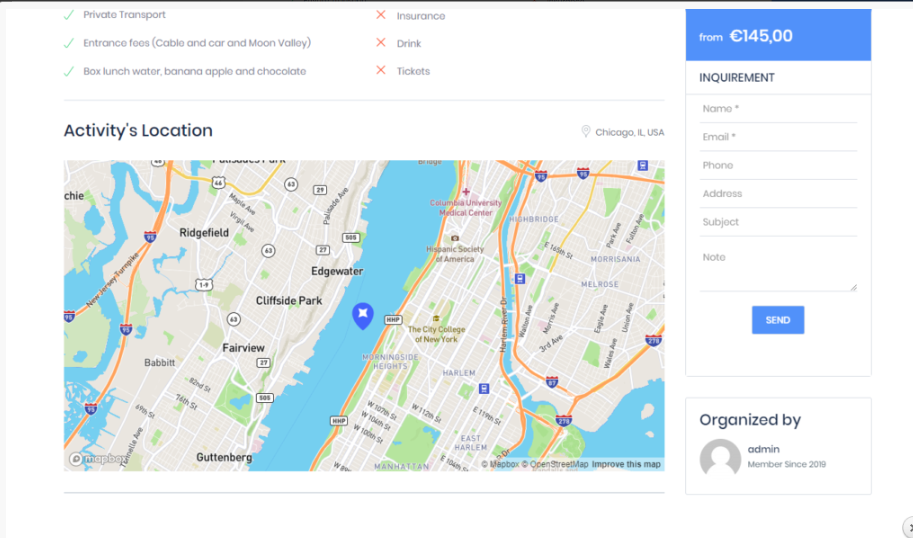This detailed map screenshot highlights various travel options within a city, primarily featuring parts of New York City, specifically Manhattan, and sections of New Jersey. 

At the top of the map, there's a checklist that includes "Private Transport" with a checkmark, followed by "Entrance Fees," "Cable and Car into Moon Valley," and provisions such as "Box Lunch," "Water," "Apple," and "Chocolate," all marked with checkmarks. Conversely, categories like "Insurance," "Drink," and "Tickets" are marked with red Xs, indicating their absence or unavailability.

To the right, in a blue bar, the amount "145,000 yen" is displayed alongside options for submitting personal information like name, email, phone number, address, subject, and a note, with a blue icon to send the information. Below this section, the text "Organized by Administrator, Member since 2019" is noted. Despite this activity being listed as located in "Chicago, Illinois, USA," the map prominently features New York City's Manhattan and surrounding areas.

The landmarks in Manhattan include the Harlem, City College of New York, and Morningside Heights. A notable blue teardrop in the river marks a "You are here" location. The map's left side shows New Jersey cities such as Ridgefield, Edgewater, Cliffside Park, Fairview, and Guttenberg. On the right, it displays parts of Manhattan, including the Harlem River Drive and Route 87. Transport icons, such as a subway symbol, and various green spaces are also visible, along with the detailed grid of streets and freeways, suggesting a comprehensive tool for exploring transportation options.